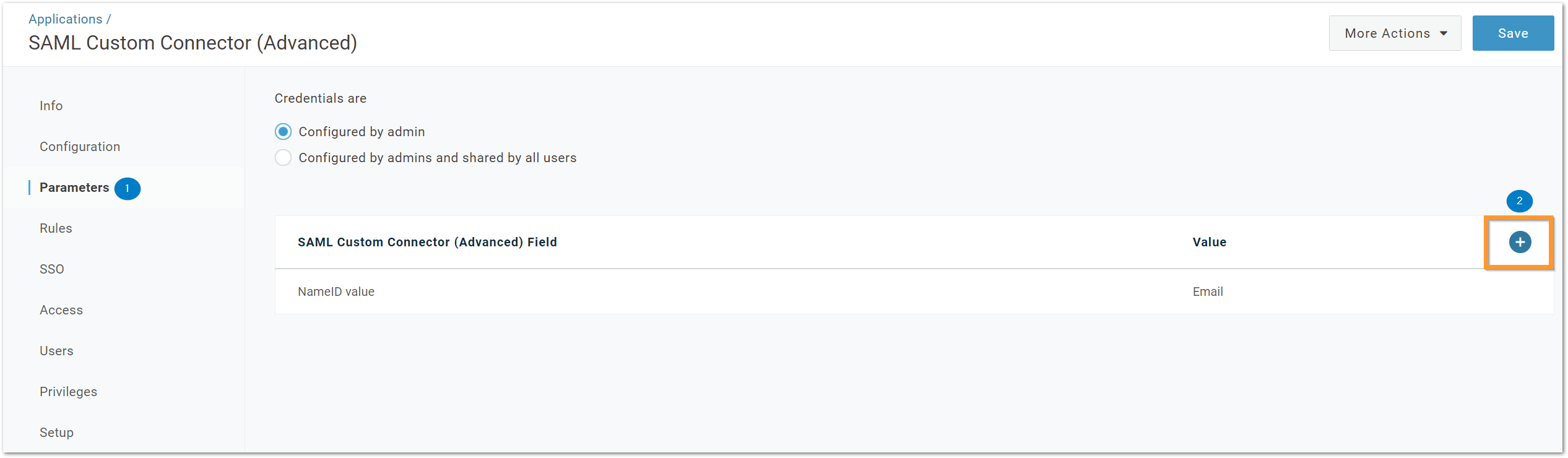The image is a detailed screenshot of a software application's interface. At the top left corner, there is a navigation link, and beneath it is the prominently displayed bold text that reads "SAML Custom Connector Advanced". To the right of this section, there are two interactive elements: a drop-down box and a blue-highlighted button.

Moving downwards to the left side of the interface, there is a navigation bar containing multiple links. The third link in the list is currently selected, indicated by a blue circle to its right and a blue line to its left, with the text highlighted in a darker, bold font.

On the right side, the interface displays text accompanied by two radio buttons, with the top radio button currently selected. Below this section, there is a chart with a single entry. Positioned to the right of the chart is a plus button, which stands out due to its orange border.